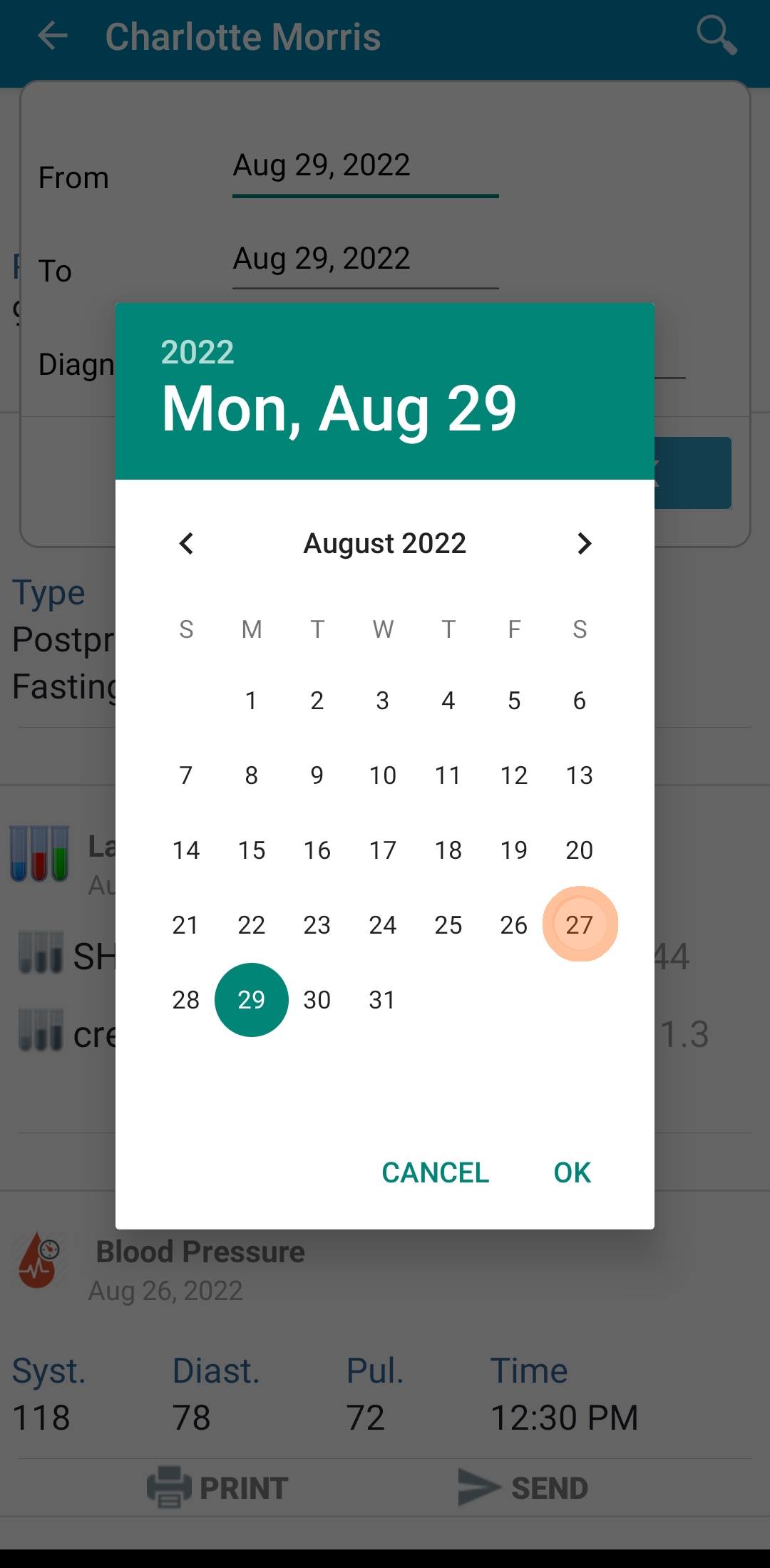The screenshot from a mobile phone prominently features a pop-up calendar interface. Centrally displayed, the calendar pop-up is framed by a box with an August 2022 calendar layout. Key details include:

- A green bar at the top showing "2022, Mulln, August 29" in white text.
- The calendar within the box highlights the 27th in orange and the 29th in green.
- At the bottom of the calendar pop-up are two green buttons labeled "Cancel" and "OK."

In the background, a greyed-out mobile page is partially visible. Details observed on this page include:

- A blue header at the top with white text reading "Charlotte Morris," accompanied by a back button and a search button.
- A section below the header that states a date range: "From August 29, 2022 to August 29, 2022."

Several elements are obscured by the calendar, but visible information comprises:

- The right edge revealing partial text "POSTP" and "FASTIN."
- A blue chart icon followed by two greyish square icons labeled "LSH" and "C."
- At the very bottom, an icon associated with blood pressure, displaying "August 26, 2022," with readings: systolic 118, diastolic 78, pulse 72, and timestamped 12:30 PM.
- Additionally, there's an icon for print or send and a thin black bar across the bottom edge of the screen.

This detailed breakdown captures the multifaceted elements presented in the screenshot, conveying both the calendar pop-up's interface and the overlapping content of the underlying mobile page.